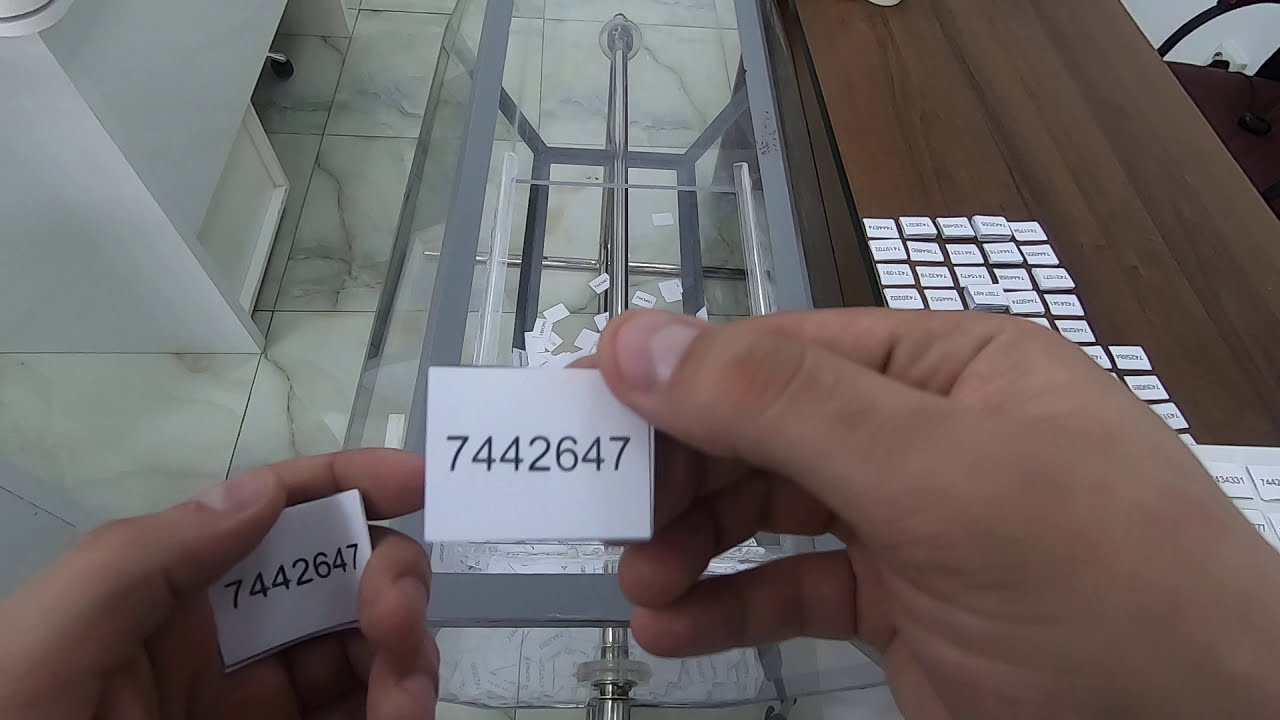In this image, we see a person sitting with both hands holding a small slip of paper, each displaying the same number: 7442647. The hands appear to be those of a man. To the right of him is a long wooden table laden with stacks of small slips of paper, though the writing on these slips is too small to discern. In front of and around him, scattered across a glass-topped surface, are more such slips of paper. By his feet, there is a see-through container brimming with additional slips and a crank mechanism, suggesting some kind of sorting or processing activity. The scene unfolds in an office setting, characterized by a white marble tile floor, part of a white desk to the left, and the wheel of an office chair just visible. The meticulous arrangement of numerically identical slips hints at an intriguing, albeit mysterious, task at hand.